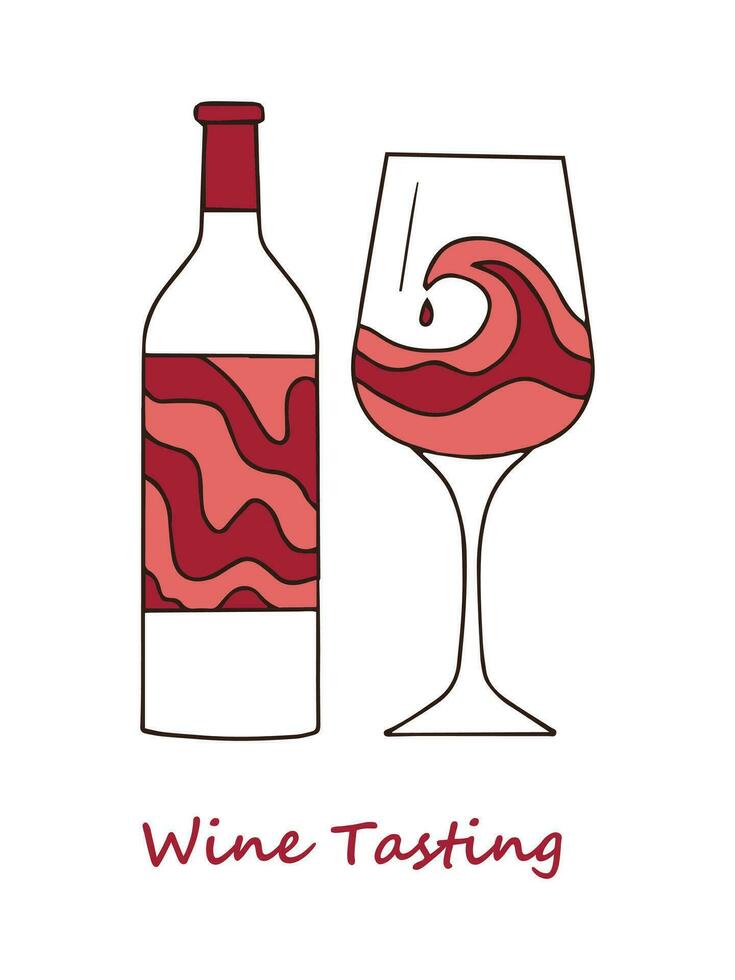In this vector-style illustration, a wine bottle and a wine glass are depicted against a white background. The bottle, positioned to the left, features a dark red cap and a red and pink label with diagonal, wavy patterns delicately outlined in black. The adjacent wine glass, nearly as tall as the bottle, contains wine that mirrors the label's hues, shaped into a dynamic wave with a single drop poised mid-fall. Below these elements, the phrase "wine tasting" is elegantly inscribed in reddish-maroon cursive. The overall composition, with its minimalist design and cohesive color scheme, evokes a sense of sophistication and fluidity, ideal for wine tasting promotions.